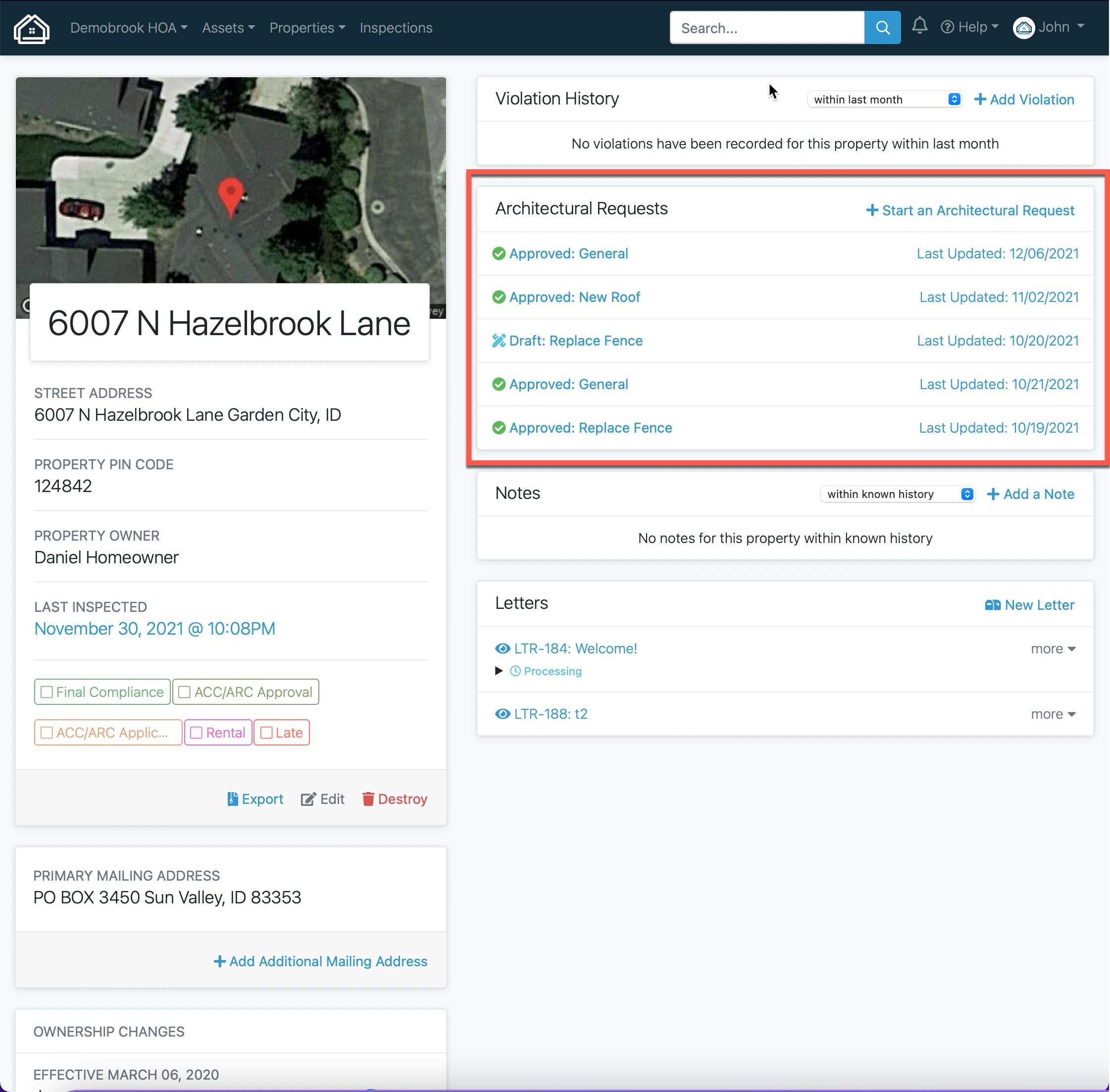The image is a square-shaped screenshot from a real estate website. On the left side, there is an aerial view map of a residence, and beneath the map, the residence's complete address, "6007 North Hazelbrook Lane," is displayed in black text on a white background. Further detailed information about the property is listed below.

The address is repeated with additional location details: "6007 Hazelbrook Lane, Garden City, ID." Below the address, the Property Identification Number (PIN), "124842," is shown in gray text, followed by the property owner's name, "Danielle Homeowner," in black text. Additional details include the last inspection date, "November 30th, 2021, at 10:08 PM," written in blue.

There is extensive information about the property, such as "Final Compliance," "ACC/ARC Approval," among other details. 

On the right side of the image, the violation history is shown in black text, followed by a section on architectural requests. Some entries in this section feature green icons with white check marks, indicating approval. Below this, there are sections dedicated to notes and letters.